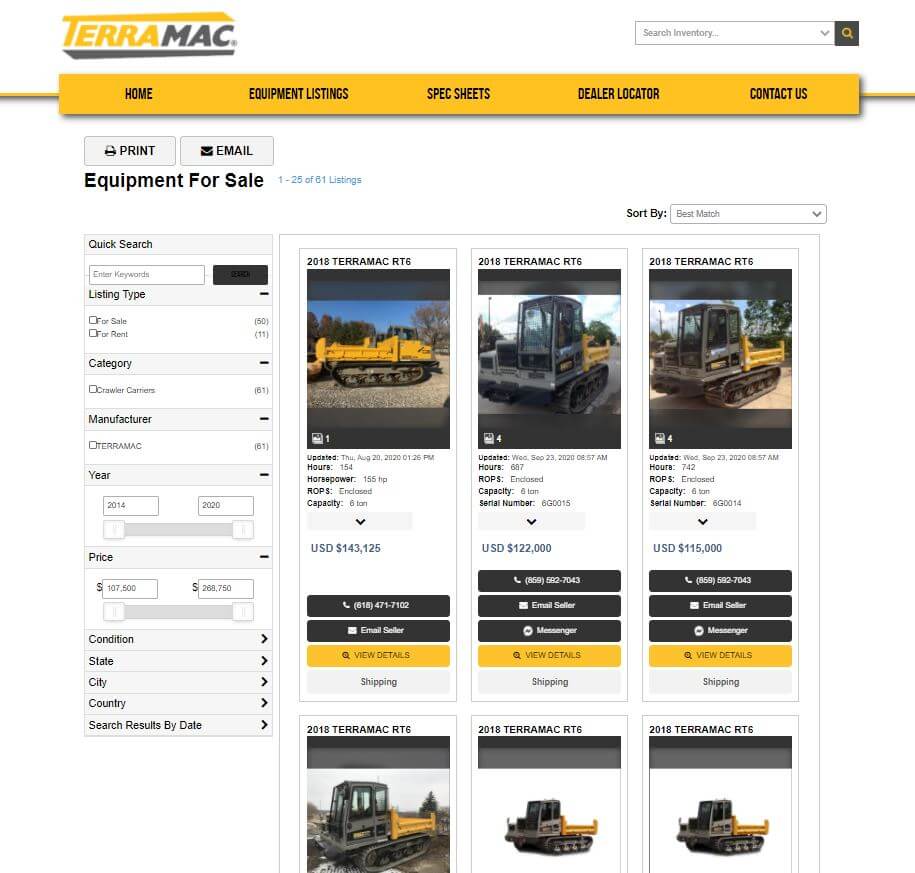Screenshot of the Terra Mac Company Website

The image captures a screenshot from the Terra Mac company's website interface. At the top of the screen, there are several navigation options displayed in a yellow bar, including "Home," "Equipment Listings," "Spec Sheets," "Dealer Locator," and "Contact Us," each accompanied by drop-down menus for further selection. Below this navigation bar, there are options to print or email the current page, alongside a prominent header labeled "Equipment for Sale."

The main section of the page is populated with rectangular boxes displaying images and detailed specifications of various construction and demolition vehicles available for purchase. Key details provided for each vehicle include the model name, horsepower, date of the last update, ROPs (Roll-Over Protection Structures) information, capacity, serial number, and price. Each box also contains options for contacting the seller via phone or email, viewing additional details, and shipping information.

The first listing features a "2018 Terra Mac RTS," and alongside it are two listings for "2018 Terra Mac RT6." Following these, several other listings are also for Terra Mac RT6 models, indicating that this specific make and model might have been a focus of the recent search query. The image, unfortunately, cuts off at the bottom, leaving some information partially obscured but still displaying pictures of the equipment.